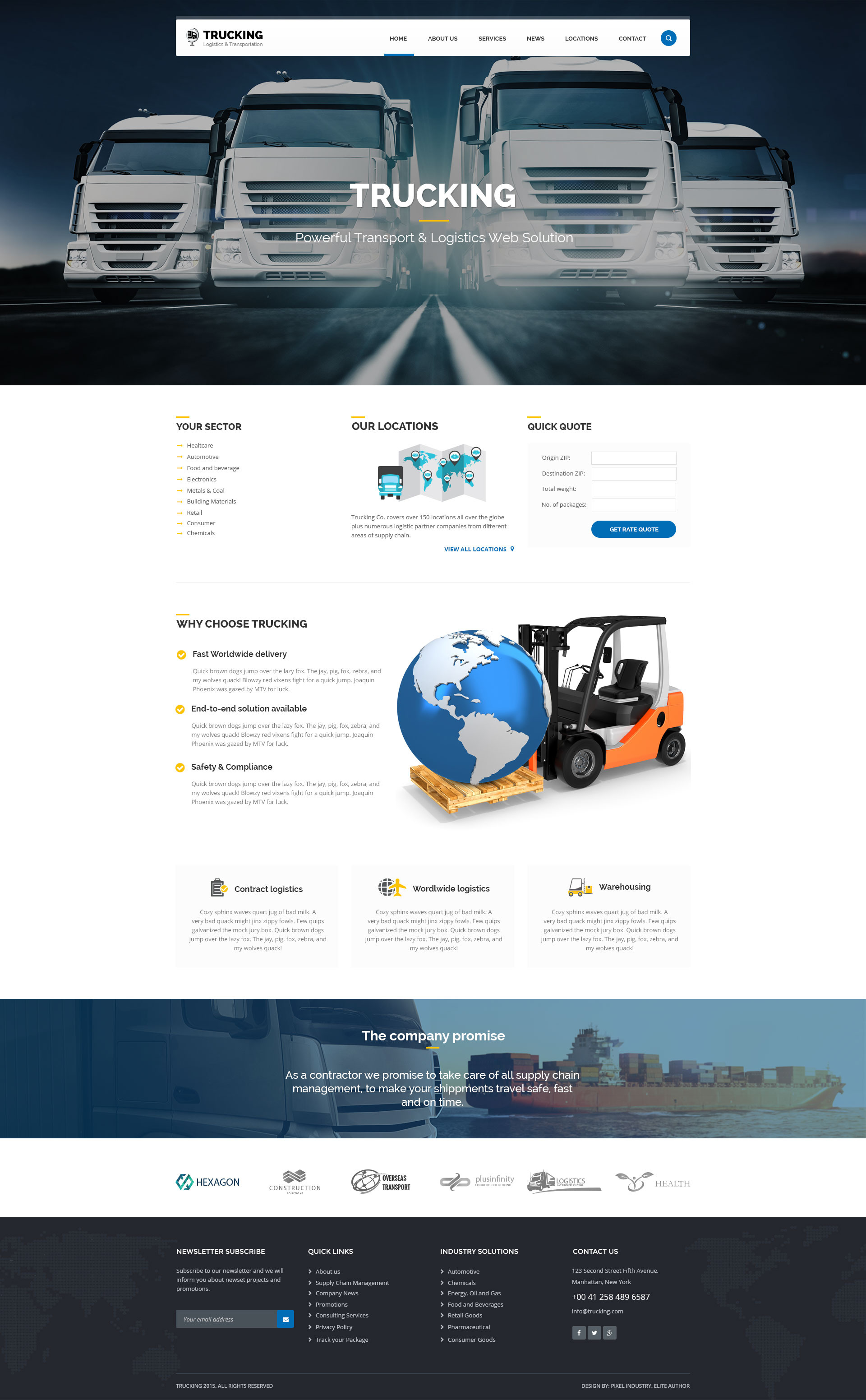The screenshot captures a comprehensive advertisement for a transport agency. The header prominently features a banner titled "Trucking," offering various selections. Just below, a striking image of four white transport trucks with darkened windows and headlights on dominates the screen, against a backdrop of a dark blue sky and lighter horizon with hills. The trucks travel down an asphalt road marked with a center line, emphasizing their journey.

Beneath this image, multiple navigation options are available. The "Your Sector" section offers diverse options, while the "Locations" center area features a small map displaying various potential locations. Adjacent to this, a "Quick Quote" section provides several selectable options. Further down, a section allows users to choose "Trucking," leading to three specific topics.

Next to this, an image showcases an orange and white forklift with black accents, seating, tires, and roll bars, lifting a pallet. The pallet supports a globe illustration displaying blue water with white landmasses, distinctly highlighting North and South America.

Below these elements are three options: "Contact Logistics," "Worldwide Logistics," and "Warehousing." Following this, a banner image displays a transport truck on one side and a large sea vessel on the other, accompanied by the company's promise statement. Finally, the bottom of the screen features various company logos, including one shaped like a hexagon, as well as additional links for a newsletter, quick links, industry solutions, and contact information.